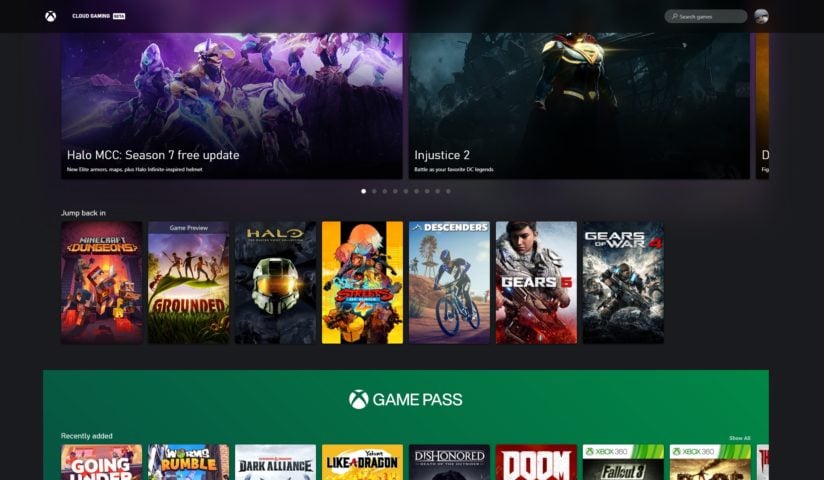The screenshot displays an Xbox interface, with an Xbox symbol prominently visible in the top left corner. The search bar, located at the top, features a magnifying glass icon followed by the text "Search game." Below the search bar is a section showcasing various games. The first game listed is "Halo MCC," specifically highlighting a capitalized "MCC" in the description, along with a mention of a new Season 7 free update. Another featured game is "Injustice 2."

To the right of these game listings, there is a grid of nine dots, with the first dot shaded white and the remaining eight in gray, indicating some form of progress or selection status. Below this section, there's a heading labeled "Jump Back In," suggesting a list of games that were previously played. The games under this category include "Minecraft Dungeons," "Grounded," "Halo," "The Sims," "Descenders," "Gears 5," and "Gears of War 4."

At the bottom of the screen is a green rectangle containing the Xbox symbol and the text "Game Pass" in white. Another section labeled "Recently Added" is visible, with an option to "Show All." From what is visible, there are eight games displayed under this recently added category.